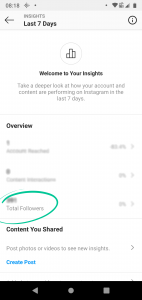The image depicts a blurry and grainy screenshot of a smartphone displaying an app interface. The page has a white background with black text at the top, reading "Insights. Last 7 days," flanked by a black arrow on the left and a help arrow on the right. Below this header, there is a centered picture of a background within a search field, accompanied by the text, "Welcome to your Insights. These are deeper," followed by unreadable text mentioning the insights from the last 7 days. 

Further down, in the middle left of the screen, there's another section titled "Overview," though the accompanying text is too blurred to read except for the line that states "Total Followers." The text "Total Followers" is distinguished by a green outline. Below this, another label reads "Content You Shared," though its description remains unreadable. At the bottom left corner of the screen, there is a blue button labeled "Create Post."